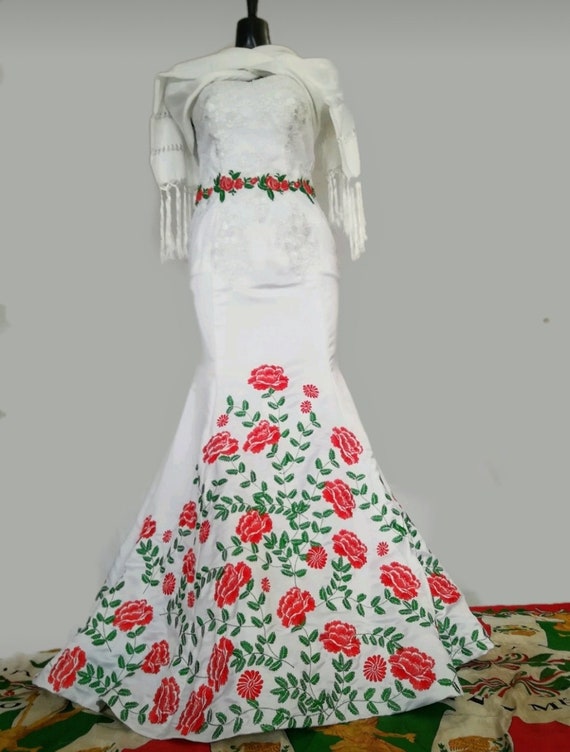The photograph features a vintage-inspired, form-fitting white dress displayed on a dressmaker's mannequin. The mannequin is identifiable by its black neck portion extending above the dress, confirming it isn't simply hanging. The dress is adorned with red roses and green leaves, especially concentrated around the waist and at the bottom, where they are more abundant and cover the flared skirt from the knees downwards. A matching narrow belt with smaller rose patterns cinches the waist. Adding to the elegance, a soft, off-white shawl with white tassels is draped over the shoulders. The backdrop is a simple white, allowing the dress to stand out. Beneath the mannequin, there is a patterned rug in red, green, and white hues, reminiscent of the Mexican flag, providing a subtle yet colorful base for the display.